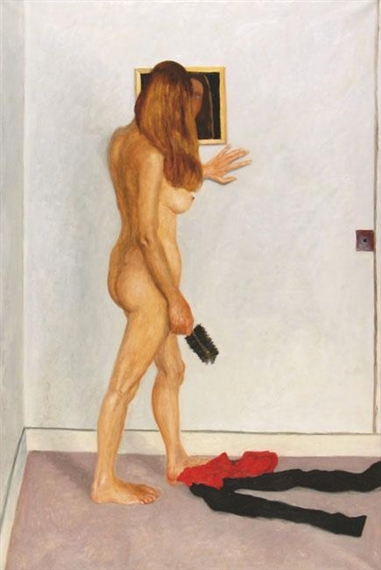In the painting titled "Mirror on the Wall, 1982" by Avigdor Arikha, a nude Caucasian woman stands in the corner of a room, facing a gray wall with her right side towards the viewer. The room's walls are a flat gray, and the floor is a peach-beige color. Scattered on the floor before her are a red garment and a black scarf, suggestive of recently discarded clothing. The woman, holding a black hairbrush in her right hand, has long golden-brown hair cascading over her right shoulder. Her left hand is placed on the wall, and her left foot is slightly extended in front of her right. Behind her, a gold-framed mirror nearly obscures a part of her reflection, notably capturing the right side of her face, which meets the viewer's gaze through the mirror. The painter employs a contemporary realist style to depict the serene yet intimate scene.